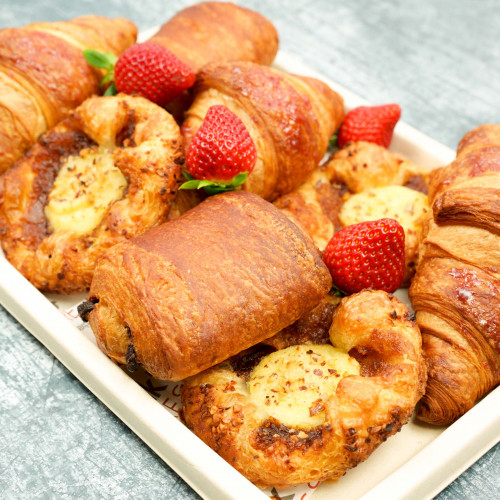This photograph features a beautifully arranged breakfast tray set against a slate-colored stone table background. The white tray, with its raised edges to prevent slipping, is laden with an assortment of delicious baked goods. The spread includes four red, juicy strawberries with their green leaves still attached, adding a fresh, vibrant touch. Among the baked items, there are four perfectly baked croissants, three delectable cheese danish bear claws, and a mouth-watering raisin apple fritter bear claw. The image captures the enticing aroma and inviting appearance of these breakfast treats, making it a feast for the eyes and the palate.